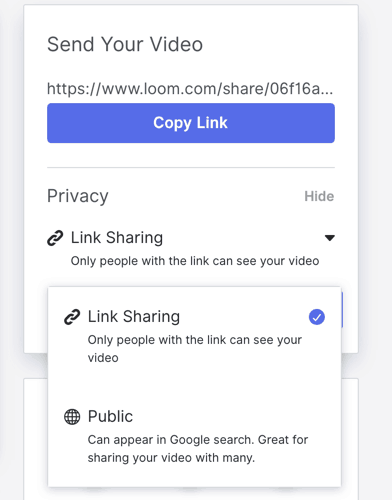The screenshot displays the interface of a link-sharing option for a video hosted on Loom. At the top, there is a URL: "www.loom.com/share/06F16a...". Below the URL, there is a blue, rectangular button labeled "Copy Link" in white text. The background behind this information is white.

To the far right of the link, there is an option for "Privacy" with a button labeled "Hide." This is followed by a section titled "Link Sharing," which features a black chain link icon. The accompanying text states, "Only people with this link can see your video," with a context button labeled "Hide" next to it, indicating it can be expanded for more options.

Further down, there is a setting showing that "Link Sharing" is checked, indicating only people with the link can view the video. Another option labeled "Public" features a round globe icon and a checkbox. The text under this option explains, "Public can appear in your Google search, great for sharing your video with many." The "Link Sharing" and "Public" options appear to be currently overlaying one another slightly in the display.